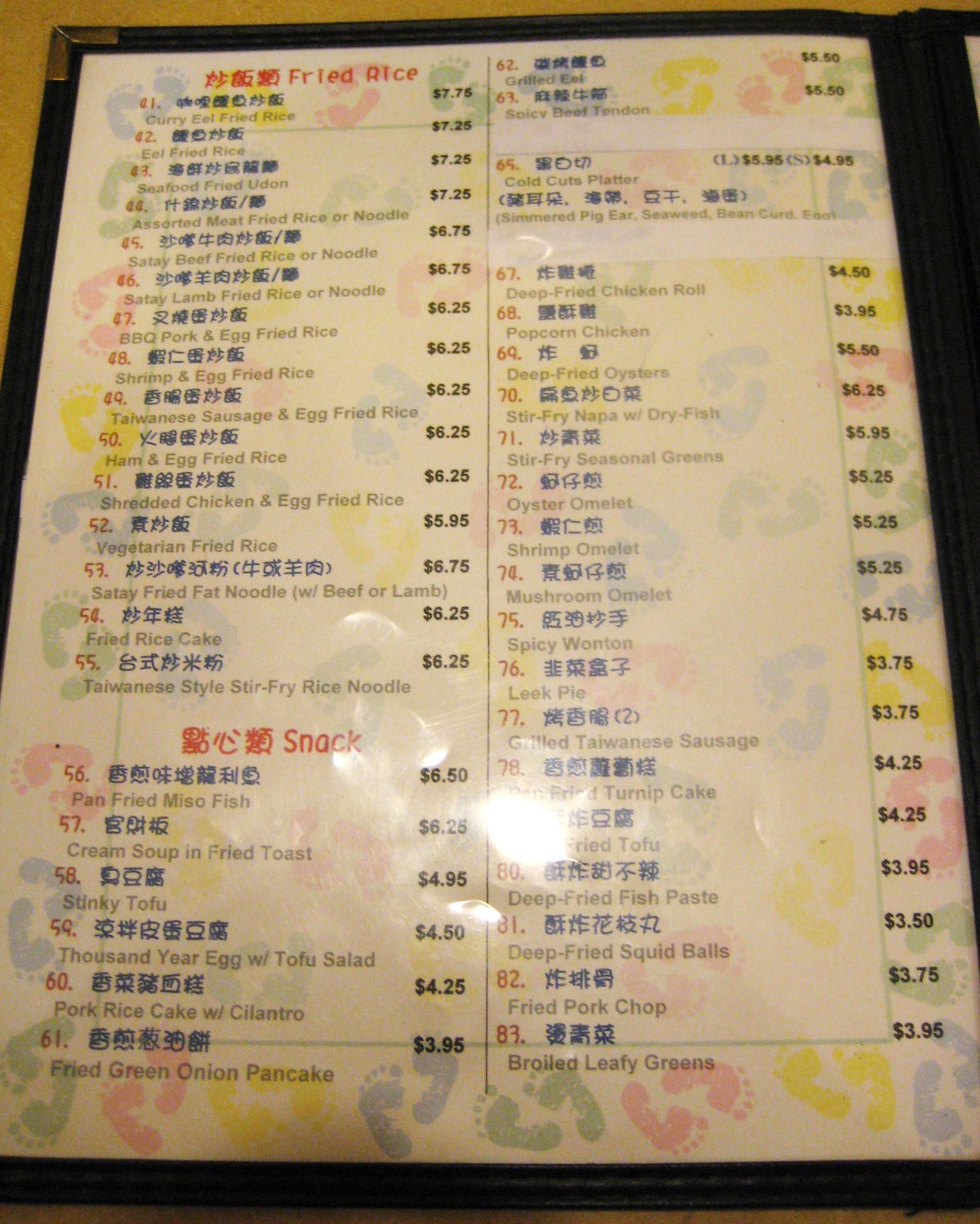The photograph captures an open page of a restaurant menu, elegantly placed on a light golden wooden table, with the wood grain visible in the upper left corner. The menu itself is encased in a black, book-style cover, offering a sturdy and sophisticated frame for the laminated, white page displayed. This page is adorned with colorful footprints—red, yellow, and blue—reminiscent of playful beach scenes, particularly around the outer edges.

The menu is dedicated to a Chinese food establishment, presenting its offerings in both Chinese characters and English. Dominating the top of the page are the Chinese characters, followed by the English title "Fried Rice" in bold red. Below this header is a comprehensive list of various fried rice dishes, each accompanied by their respective prices, predominantly in the $6 range. Though some items at the top of the page are out of focus, the middle section clearly features options such as "Taiwanese Sausage and Egg Fried Rice," "Shredded Chicken and Egg Fried Rice," and "Vegetarian Fried Rice." The menu also hints at an assortment of snacks and other culinary delights yet to be explored on adjacent pages.